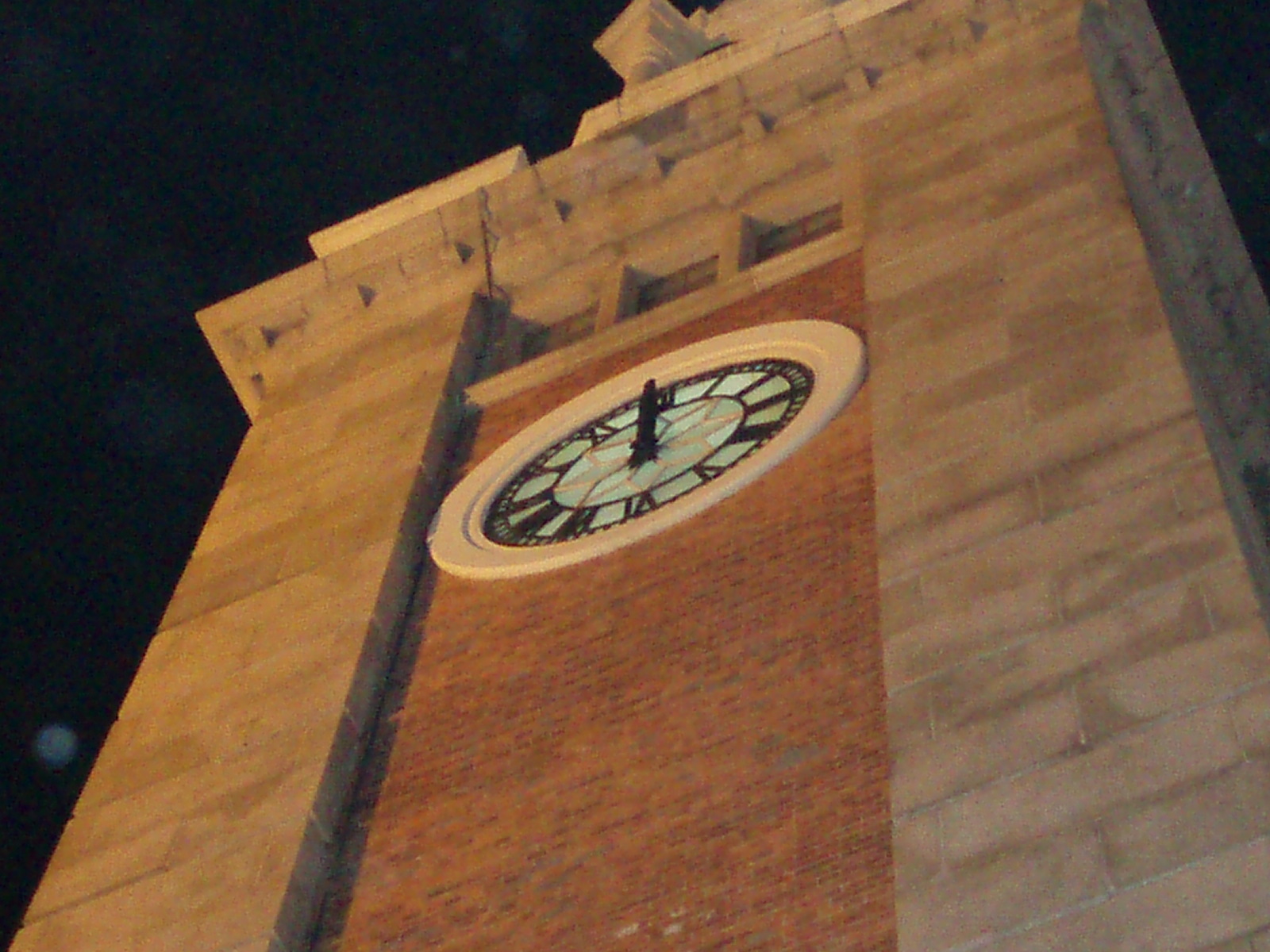The image showcases an imposing clock tower, captured from a low-angle perspective that accentuates its grandeur. Dominating the center is a clock face reminiscent of London's iconic Big Ben, adorned with elegant Roman numerals. The structure is primarily constructed of tan bricks, with a striking section of red brick encircling the clock. The backdrop is a deep, velvety black, punctuated by subtle white orb reflections, which may suggest either an artistic effect or light reflections. The clock reads exactly 12 o'clock, creating a sense of timelessness or a moment frozen in time. Above the clock, intricate stone and pillar details contribute to the tower's majestic appearance. The overall composition blends elements of historical architecture with a touch of modern artistic flair.